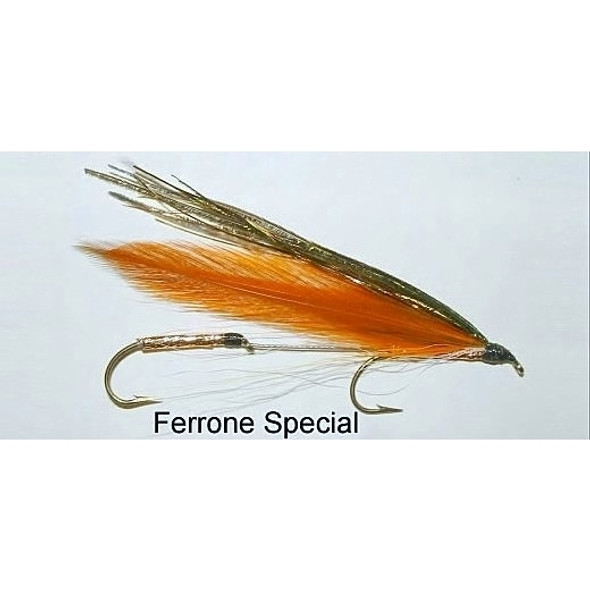The image is a close-up, color photograph of a fly fishing lure positioned at the center of a rectangular frame. The backdrop is a bluish-gray hue, providing a neutral contrast to the lure. The fishing lure itself features a metallic silver base with two curved hooks extending downward and to the right, complete with small barbs near their tips. At the front of the lure, there's a small metallic loop designed for attaching a fishing line. 

Adorning the lure are two prominent feathers: a vibrant, bright rusty orange feather positioned centrally, and a metallic green feather rising above it, giving the lure the appearance of a bug or dragonfly. The text "Ferron Special" is displayed in black lettering at the bottom of the image, just below the hooks. The colors of the lure include shades of gray, brown, orange, brass, silver, and black, creating a visually striking and detailed product suitable for a sporting goods site.